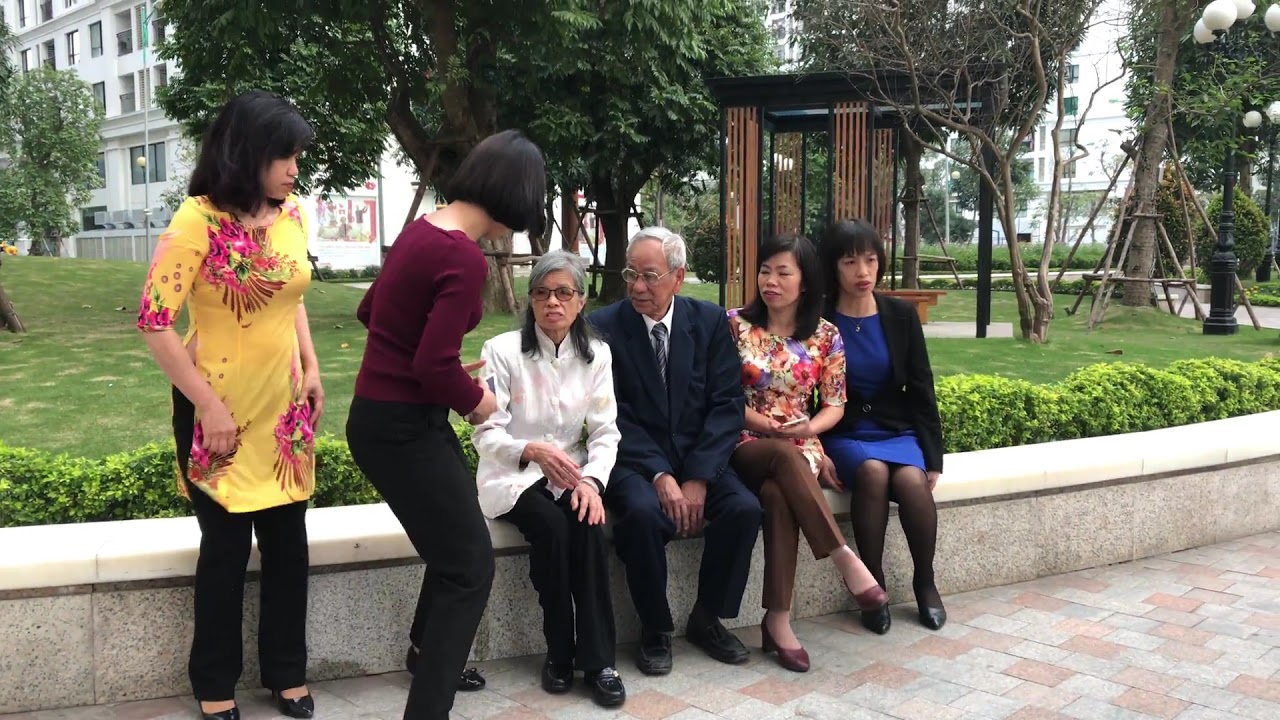In this vibrant outdoor family photo set against a scenic park with shrubbery, well-trimmed bushes, and a brick-tiled walkway, we see an Asian family arranged near a stone wall with a flat white top. Central to the image are an elderly man in an all-black suit with a white shirt and tie, and an elderly woman in a white shirt and black dressy pants. These look like the parents or grandparents, sitting together on the stone ledge.

Flanking them on either side are what appears to be their family members—four females and one male. Three women and the man are seated next to the elderly couple: one woman sports a colorful yellow dress with red flowers over black dressy pants and black shoes, another wears a dark burgundy sweater with black pants and shoes, while the third woman has an overall dress adorned with a myriad of colors, including white, red, purple, and orange over brown dressy pants and shoes. The fourth female, decked out in a blue dress paired with black stockings, shoes, and a black jacket, and a second woman are standing and conversing, the former with her side turned mostly away from the elderly woman.

In the backdrop, the well-maintained park features a lush green lawn, trees, and small gazebo-like structures, encapsulating a serene and familial atmosphere. The family looks engaged in conversation, possibly organizing themselves for a family portrait.